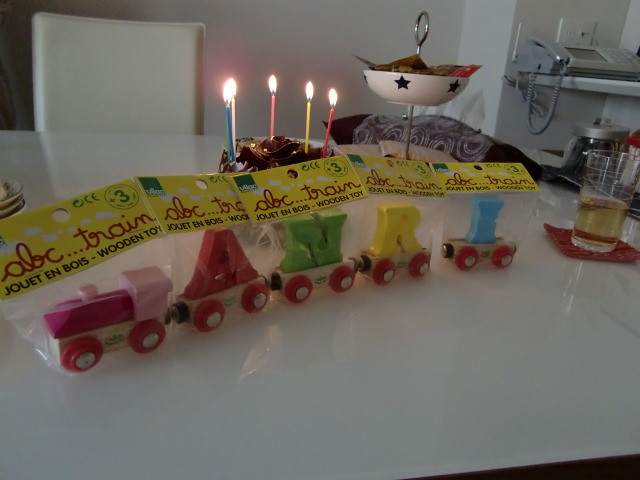In the image, there is a detailed arrangement on a white tabletop. Central to the scene is a chocolate birthday cake, adorned with five colorful lit candles in blue, white, pink, yellow, and red, each glowing with a yellow flame. In front of the cake, a packaged wooden ABC train is displayed, with individual letters on the train cars spelling out "A-N-R-I," each part of the train connected by magnets. The train has letters in red, green, yellow, and blue. Also on the table, to the right of the train, is a clear plastic cup containing a liquid and placed on a red napkin. In the background, to the left, there is a white chair. To the right, there is a set of shelves next to an outlet, with various items including a glass container with a silver lid and a gray telephone. Additionally, there is a dish with some items on it placed next to the cake. The scene exudes a festive yet organized appearance, with the white table providing a clean backdrop for the vibrant items displayed.